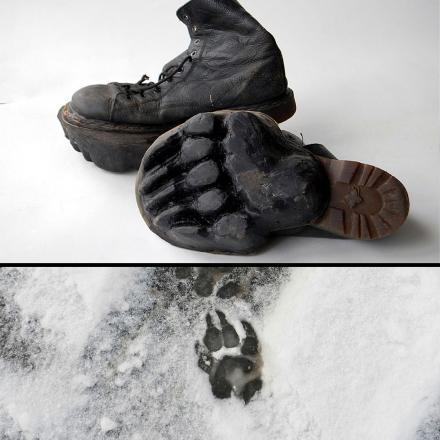The image consists of two full-color photographs: the top one is square, and the bottom one is horizontally rectangular. They are separated by a thin black line. In the upper photograph, there are two very old, worn black leather boots. One boot is lying on its side, clearly displaying its sole, while the other stands upright. These boots have been modified, with the front part of the soles designed to resemble a large animal's clawed footprint. The bottom photograph shows a light dusting of snow on the ground featuring a single, large animal footprint with visible claws. The similarity between the modified boot soles and the footprint in the snow suggests that someone walked through the area wearing these specially altered boots, creating the illusion of a wild animal having passed by.